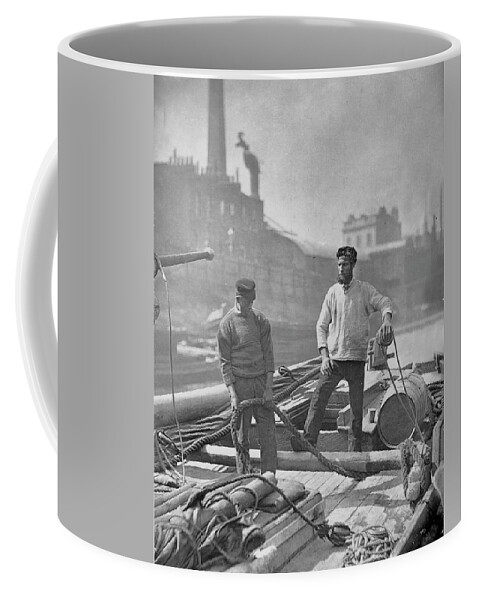The coffee mug boasts a sleek white handle, lip, and a gray interior. The exterior of the mug features a professional grayscale image, which is a striking black, white, and gray depiction of two bearded men standing on wide-planked wooden flooring. The scene appears to capture a moment on a docked boat or barge, with various barrels and thick ropes around them. One man, wearing a long-sleeved shirt, hat, and pants, is holding a rope and looking down, while the other man, dressed similarly, gazes at him. Behind them, an industrial backdrop of factories and buildings, complete with billowing smoke from a chimney, sets a dramatic scene underlined by the historical feel of the image. The dominant white background of the mug further accentuates the overlaid artwork, creating a visually appealing product.